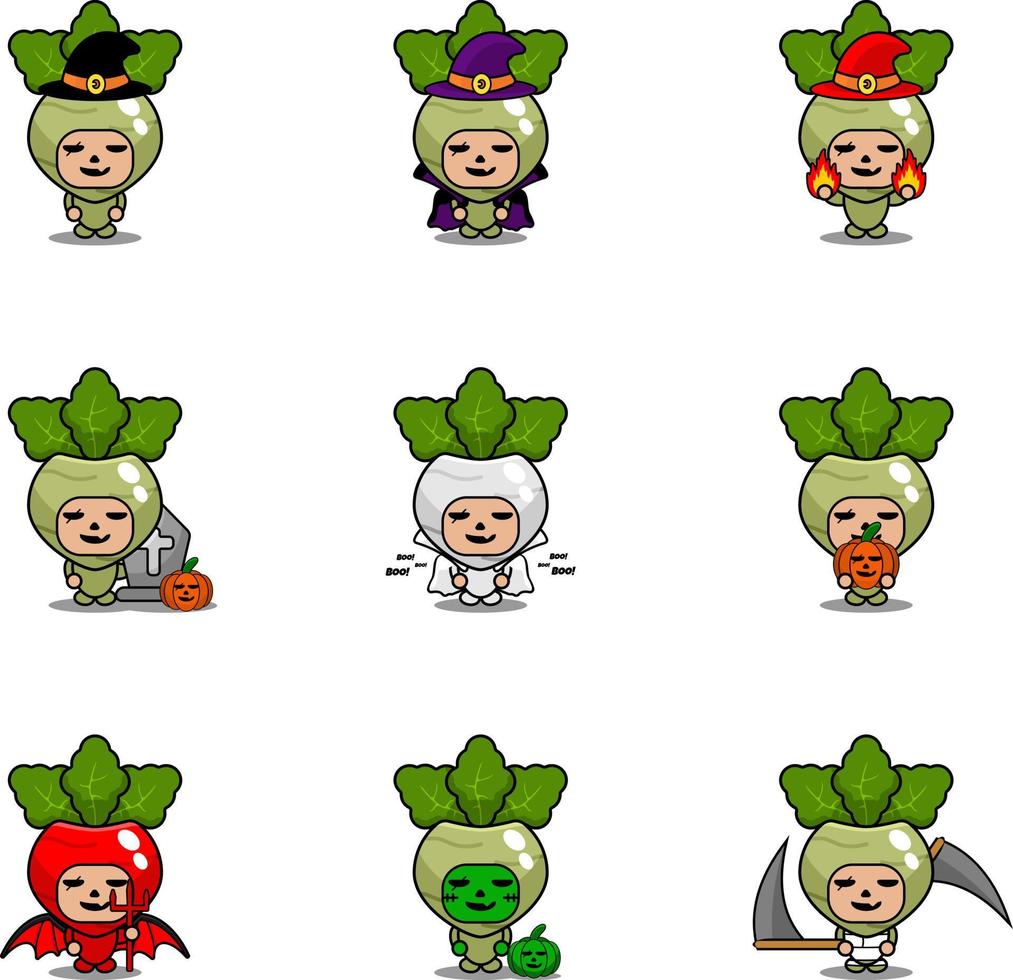The image showcases a grid of nine cartoon vegetable characters, each resembling a turnip with a jack-o'-lantern face. The characters, displayed in a 3x3 format, stand against a white background and wear various Halloween-inspired costumes. They don witch hats in black, purple, and red, with some characters carrying carved pumpkins or standing beside graves. Other costumes include a zombie, a devil with a pitchfork, a ghost saying "boo," and one holding dual sickles. Each character features leaves sprouting from the top of their heads, enhancing their whimsical vegetable personas. The costumes and accessories display themes of Halloween such as Dracula, zombies, witches, and devils, using vibrant colors like red, purple, black, and green.